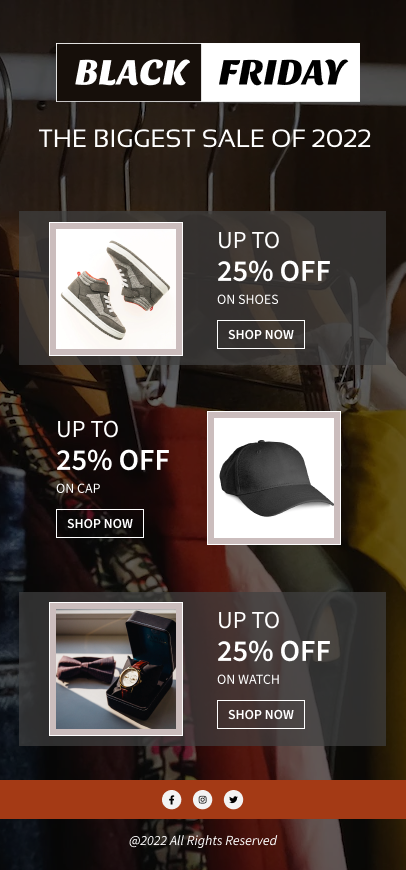**Descriptive Caption:**

This screenshot captures a vibrant Black Friday promotional flyer displayed on a mobile phone screen, highlighting the biggest sale of 2022. The heading "Black Friday" is split into two contrasting sections: "Black" appears in striking white letters against a black background, while "Friday" features a harmonious white-on-white theme.

Below the headline, the flyer showcases enticing sale items and discounts:

- **Tennis Shoes:** A pair of trendy sneakers is prominently featured, with a label indicating "Up to 25% off on shoes". A call-to-action "Shop Now" encourages immediate engagement.
- **Baseball Cap:** Positioned beneath the shoes, a standard yet stylish black baseball cap is advertised with the same "Up to 25% off on cap" discount and "Shop Now" prompt.
- **Watch:** A sophisticated watch encased in a box, paired with an elegant bow tie, suggests a classy accessory option. The consistent "Up to 25% off on watch" discount and "Shop Now" button are also visible.

A distinctive red banner runs horizontally along the bottom of the screen, adorned with icons for social media platforms Facebook, Instagram, and Twitter, inviting users to subscribe and stay informed about ongoing sales and events.

The footer notes include a "© 2022 All rights reserved" disclaimer. The backdrop of the image features a clothing rack filled with an assortment of garments, indicating that the department store offers a wide range of clothing items in addition to the highlighted products.